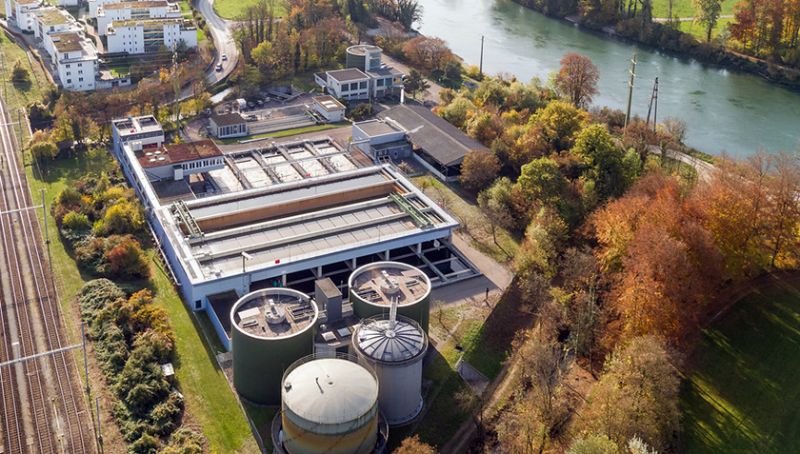This aerial photograph depicts a processing plant or factory prominently positioned in the center, featuring a large square-shaped central building likely constructed from materials such as cement or stone. The building is accompanied by four cylindrical silos, possibly utilized for loading and unloading materials via the adjacent train tracks running along the left side of the image. The factory is surrounded by dense foliage showcasing a range of fall colors—golden orange, red, yellow, and brown—indicating that the photo was taken in autumn. In the top-right portion of the image, there's a gently flowing, greenish canal. To the left, several smaller structures and what appear to be apartment buildings are visible. Further adding to the detail, a highway with light traffic curves around the background, and power lines can be seen near the water on the top right. Additionally, the image includes some white signs on or next to the central building, underscoring the industrial setting. The overall color saturation of the image is low, giving it a muted, autumnal feel.